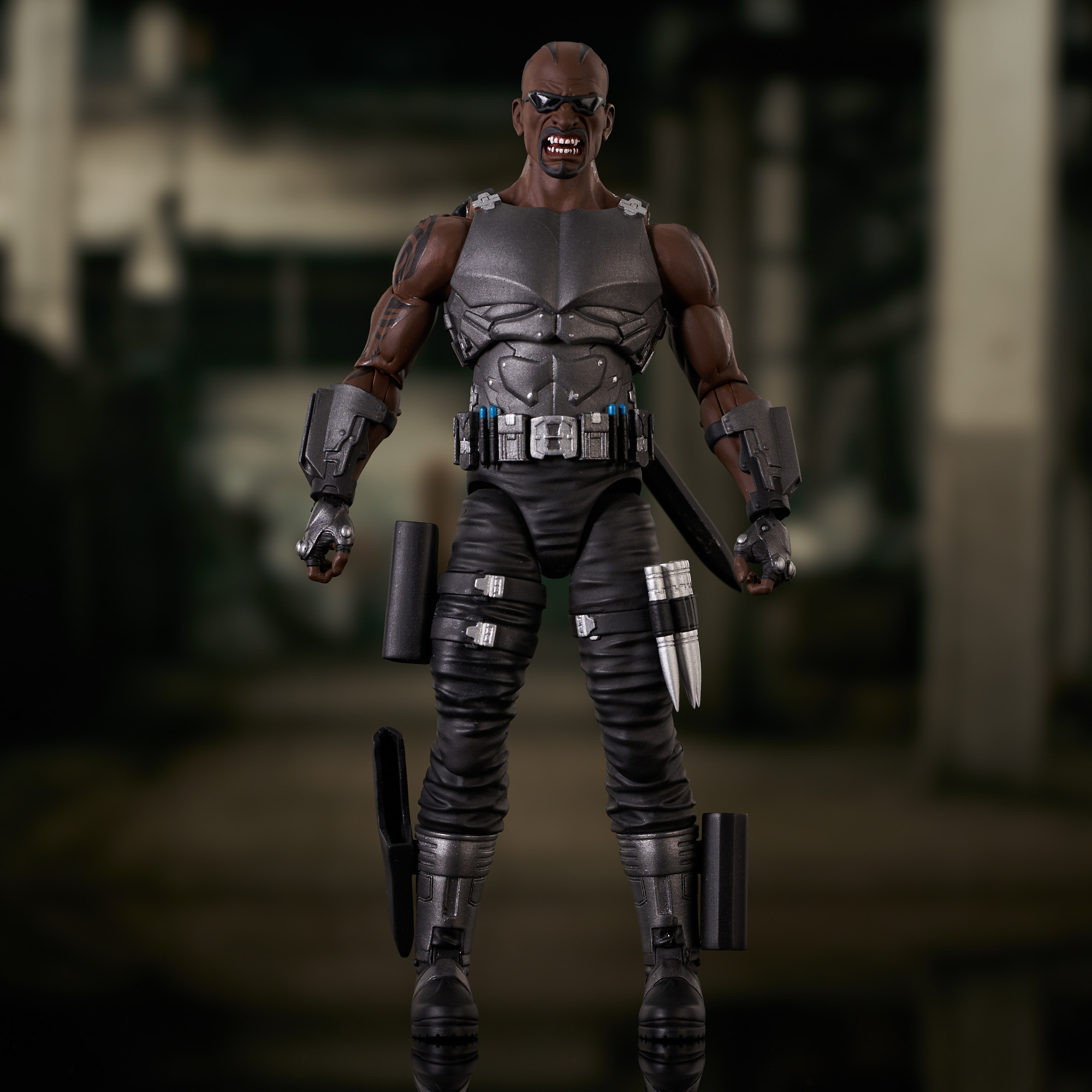In this highly detailed close-up photograph, we see an action figure that represents an African-American character with dark skin. His head is bald, adorned with two black tattoos or stripes, and his eyes are shielded by sunglasses. His facial expression is fierce, with his mouth wide open in a menacing snarl, displaying a full set of white teeth.

The action figure is outfitted with elaborate gear and weapons. He wears a grey, metallic chest armor covering his torso, and his forearms are protected by mechanized gauntlets. Both his arms also feature tribal-style tattoos, adding to his intimidating appearance. His hands are gloved, and a utility belt encircles his waist, filled with various tools and weapons that are silver, black, and blue.

He dons skin-tight black leather pants, strapped with ammunition on both thighs. His tall, steel-toed boots are similarly accessorized; the left boot has a black box while the right one includes a knife sheath. Additional weapons, possibly a nightstick or flashlight, are attached to his boots, signaling his preparedness for battle.

The background suggests an industrial or factory setting, likely digitally inserted, placing the action figure in the midst of what appears to be a gritty, urban environment. The figure stands poised, ready for action, embodying the essence of a superhero or DC character.